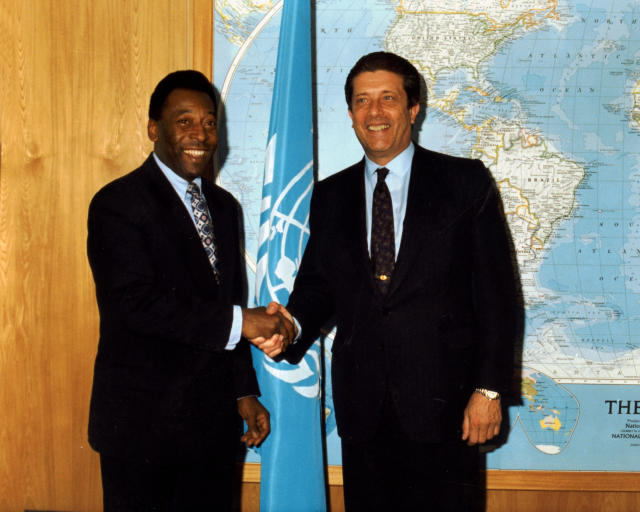This photo features the legendary soccer player Pelé, standing on the left, shaking hands with a Caucasian gentleman on the right. Both individuals are dressed in black suits and blue undershirts, exuding an air of importance and dignity. Pelé's ensemble is completed with a white tie adorned with blue and orange circular designs, while his counterpart sports a brown tie featuring a gold dot near the bottom. 

A wristwatch peeks out from beneath the man's jacket sleeve. They are both smiling warmly, emphasizing the friendly nature of their meeting. The setting includes a light brown wooden wall with a trim visible at the bottom. Behind them, a large world map is mounted on the wall, and a light blue and white flag hangs on a pole positioned directly between the two men. The style of their attire suggests that the photograph might date back to the mid-80s to early 90s.